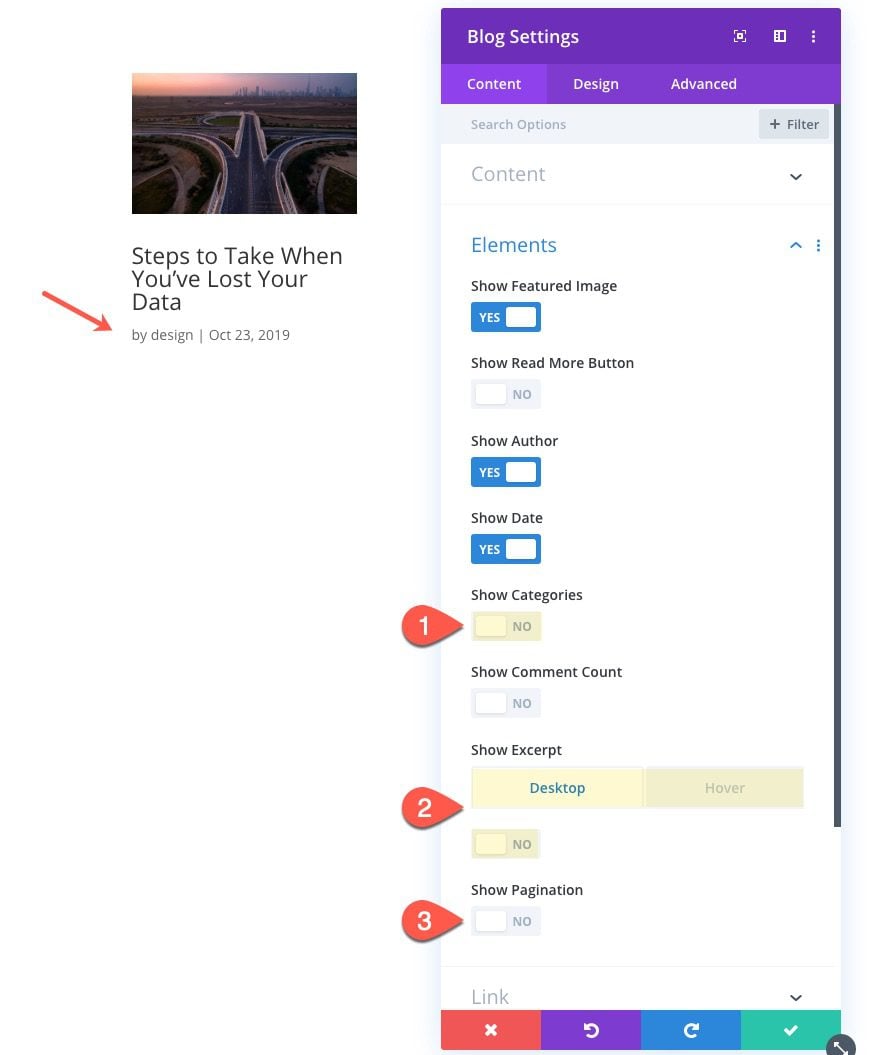The image consists of two main sections. In the upper left corner, there is a small rectangle showcasing a road that splits into two, heading left and right. Beneath this visual, the text reads, "Steps to take when you've lost your data." A red arrow points towards the phrase "by design October 23rd, 2019."

At the top, a large, narrow purple rectangle displays the text "Blog Settings," along with three tabs labeled "Content," "Design," and "Advanced," with the "Content" tab selected. Below these tabs, there are several toggles under the "Elements" section: 

- "Show featured image" is toggled to yes.
- "Show read more button" is set to no.
- "Show author" is toggled to yes.
- "Show date" is toggled to yes.

Additionally, the "Show categories" option is marked with a number one indicator and is currently set to no. 

Further down, the "Show comment count" option is also set to no. The "Show excerpt" option, which has a desktop-specific setting, is highlighted by an orange number two indicator. Lastly, the "Show pagination" option is marked with a number three bubble and set to no.

At the bottom of the image, navigation icons include a red X, a purple arrow pointing left, a blue arrow pointing right, and a green checkmark.